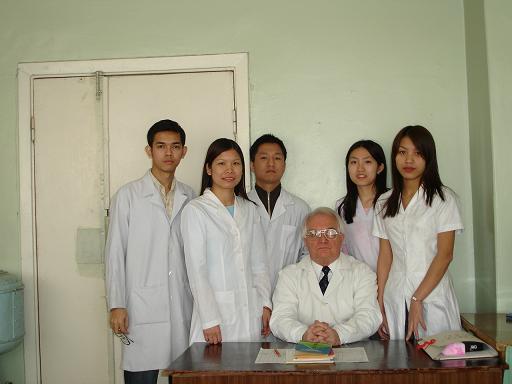In this photograph, we see a group of six medical professionals, five younger individuals, and an older gentleman who appears to be their professor or supervisor. The older man, with pale skin and very short white hair, is seated at a desk, wearing a white lab coat over a white collared shirt and dark tie. His hands are neatly clasped on the desk, which is cluttered with paperwork, a notebook, a longer piece of paper, and a red pen to his right. On his left, there is a fancy folder tied with a red ribbon, filled with thick papers, some pink and some black.

Behind him stand five younger colleagues or students, all dressed in white lab coats. Starting from the left, the first individual has tan skin and appears masculine. Next to him is a feminine-presenting person with pale skin and long dark hair. The third and middle individual, masculine with very short hair and dark tan skin, is slightly in the back and wears a dark collared shirt under their lab coat. The fourth person has very long hair and paler skin. Finally, the fifth individual, to the far right, has dark brown hair and medium tan skin. The group stands in a rather dull gray room with a white door in the background, next to which is a water cooler.

The overall setting is an austere office, possibly within a hospital or medical facility, indicated by the presence of a sterilizing unit near the door. All six individuals are looking at the camera, most of them smiling, capturing a moment of professional camaraderie.